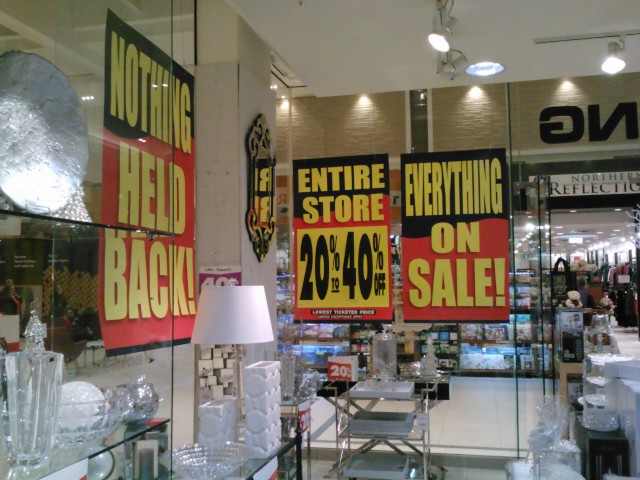The image depicts a section of a store, possibly taken towards its entrance. On the right side of the image, the entrance signage of a neighboring store named "Northern Reflections" is visible, though the letters "G" and "N" appear reversed. In the foreground, glass shelves display an array of crystal jars, bowls, and white lamps, contributing to a predominantly white aesthetic.

Large, eye-catching posters in black and red with yellow text dominate the scene. One on the left reads "Nothing Held Back," while another on a glass panel in front states "Entire Store." Below this, black text on a yellow background advertises a discount range of "20% to 40% Off." Another poster further emphasizes that "Everything On Sale," positioned above an additional display.

In the background, beyond the store's confines, a glimpse of another store across the hall can be seen, lined with numerous books or magazines, adding depth to the composition.